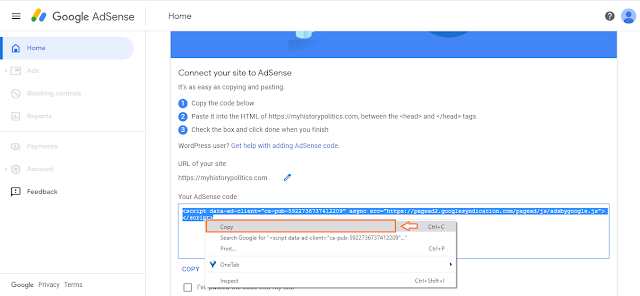Here is the cleaned-up and detailed caption for the screenshot:

---

The screenshot showcases the Google AdSense dashboard. On the left sidebar, the column header reads "Google AdSense," with a three-line hamburger menu icon positioned to its left. The sidebar features several navigational options. The "Home" option is currently selected, marked by darker blue text and a pill-shaped light blue highlight. Below "Home," there are grayed-out options listed sequentially: "Ads," "Blocking Controls," "Reports," "Payments," and "Account." At the very bottom of the column is the "Feedback" option in black text.

To the right of the sidebar is the main content area for the home menu. At the top of this content area, a long blue bar spans the width of the window. Beneath this bar is a white background containing black text that instructs, "Connect your site to AdSense. It's as easy as copying and pasting." The steps to connect the site are illustrated below, represented by three dots, each within small blue circles containing white text labeled "1," "2," and "3."

The specific steps are as follows:
1. Copy the code provided below.
2. Paste it into the HTML of https://myhistorypolitics.com between the <head> tags.
3. Check the box and click "Done" when finished.

---